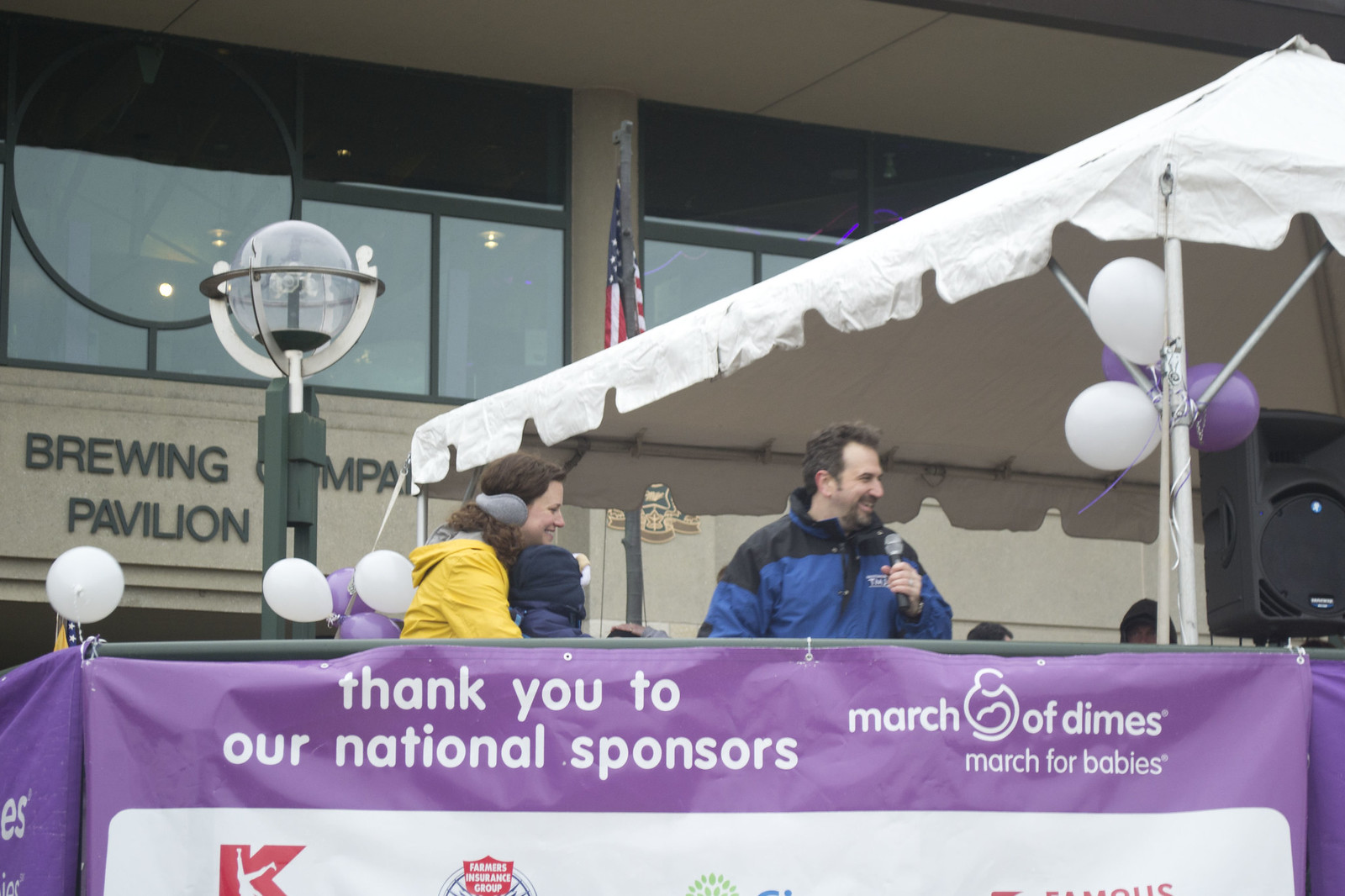The image depicts an outdoor event, likely a parade or a race, featuring multiple people standing on a raised stage covered by a rectangular cloth tent canopy upheld by several white poles. To the right of the stage, there is a speaker setup. In front of the stage, a metal railing displays multiple purple banners secured with zip ties. One prominently visible banner reads, "Thank you to our national sponsors, March of Dimes, March for Babies," and shows a white rectangle with partially visible logos. In the background, there is a rectangular building with large glass panes. Part of the building made of stone bears black lettering that reads "Bring." Central to the image is a man wearing a blue jacket, holding a microphone, and smiling, standing beside a woman in a yellow shirt who is hugging a child. Both appear to be engaged with the activities on stage.